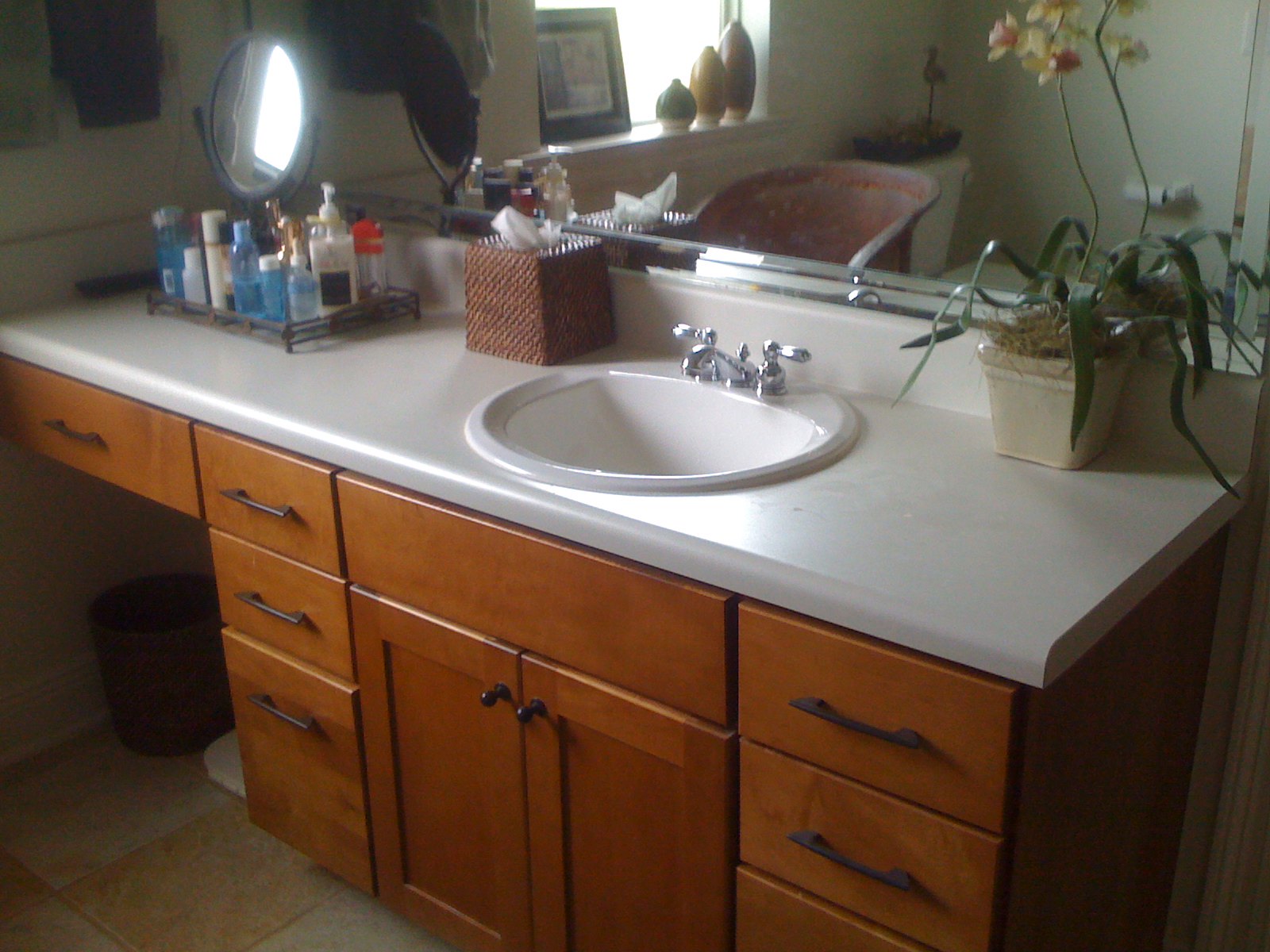The bathroom is elegantly designed, featuring pristine white tiled walls and a sunken white porcelain sink. The sink is complemented by sleek silver knobs and a matching silver faucet, all of which appear spotless. Below the sink, there is a chestnut wood cabinet with ten compartments, adding both functionality and warmth to the space. The floor is tiled in a mix of beige and white, providing a neutral backdrop. A small black trash can is tucked neatly beside the cabinet. The countertop is adorned with an assortment of soaps, skincare products, and other accessories, indicating a well-cared-for personal space.

Above the sink, a gleaming mirror reflects light beautifully, further enhancing the room's brightness. Unconventionally, a pink chair is placed in the bathroom, offering a place to sit, perhaps for a leisurely grooming routine. The chair sits in front of a small desk that holds a vibrant green plant and a picture frame, adding a touch of personalization and comfort to the room.